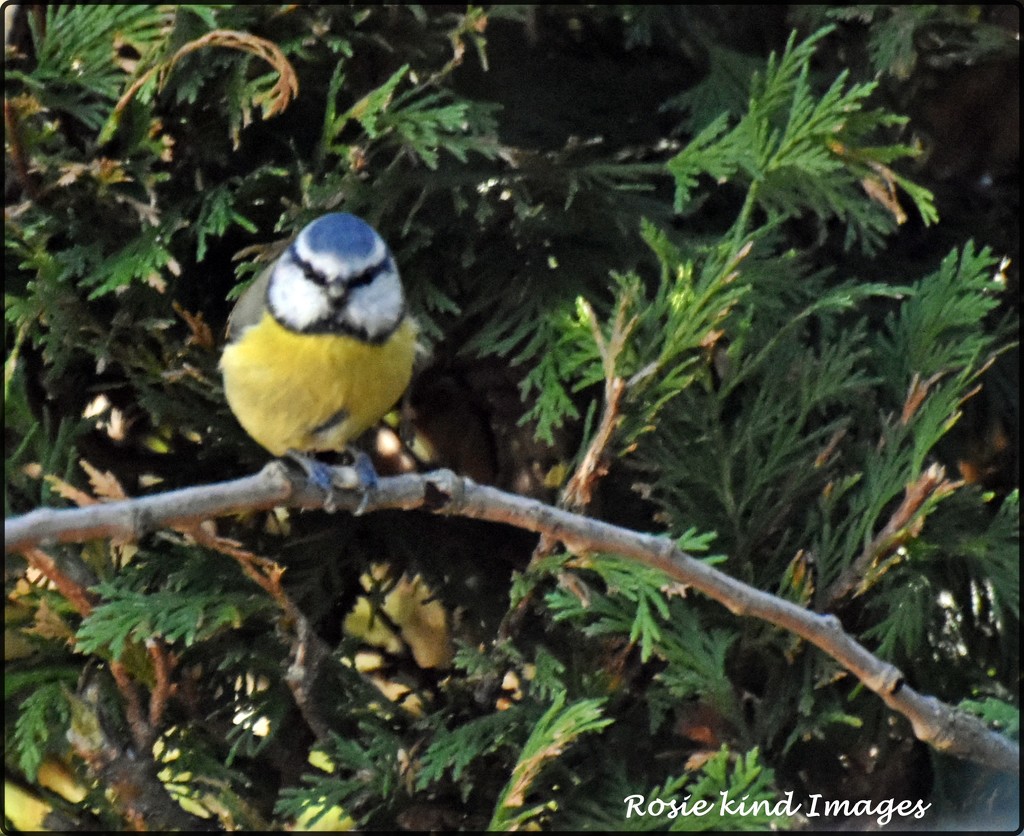In this detailed photograph taken outdoors, we see a striking bird perched atop a slender, curved brown branch that stretches across the foreground. This lone avian features a prominent bright yellow belly, a white face marked with black bands resembling goggles across its eyes, and a bluish crown adorning its head. Its short beak and black talons grasp the thin branch firmly. The background is filled with a dense, green foliage that appears to be from an evergreen or arborvitae tree, creating a lush and natural setting. Notably, white text at the bottom right of the image reads "Rosy Kind Images," indicating the photographer or the company behind this captivating shot. The close-up view highlights the bird’s vivid colors and markings, making it the focal point against the verdant backdrop.